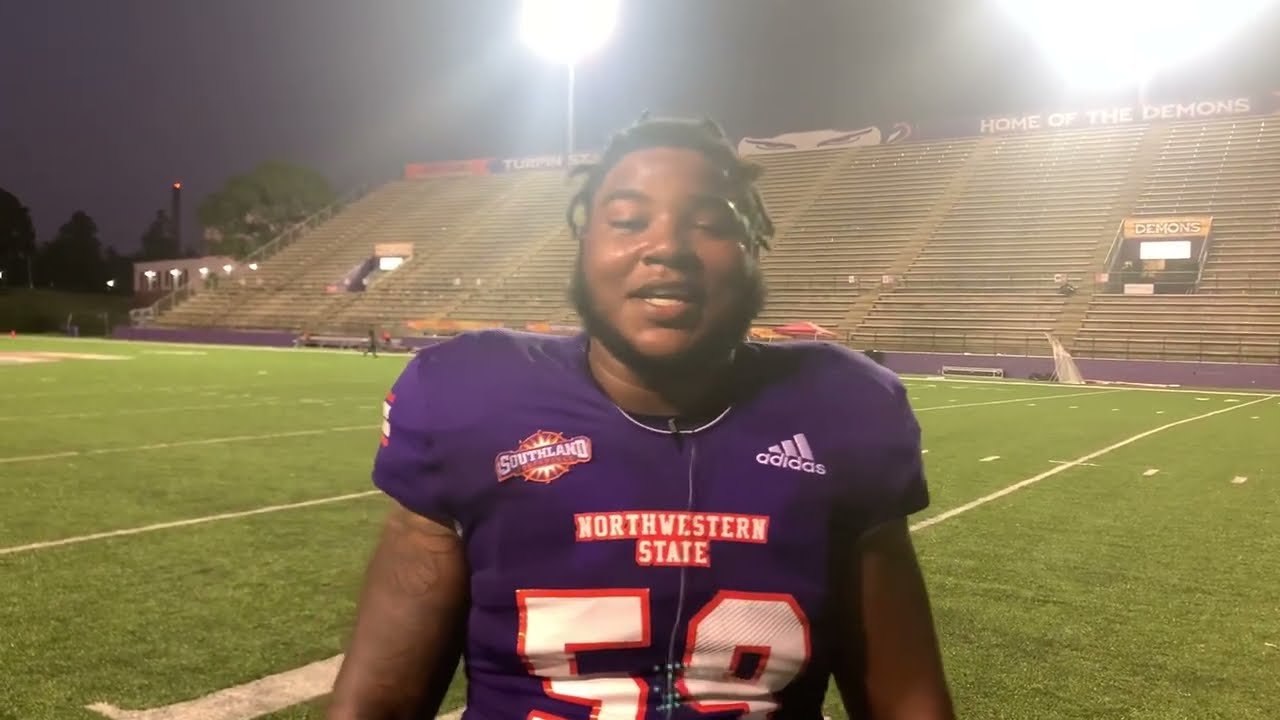In this captivating photograph, an African-American football player stands on a green football field under the vibrant glare of stadium lights, casting bright reflections through the dark night sky. The smiling player, with black short dreadlocks and a beard, appears to be engaging in conversation, his eyes half-closed and teeth visible. He wears a purple Northwestern State jersey with the number 59 prominently displayed in bold white letters outlined in orange. The jersey also features an Adidas logo on the right chest and a Southland Conference emblem on the left. Behind the player, grayish-tan bleachers with a blue wall in front sit empty under the sign "Home of the Demons," and trees are visible on the left edge of the image, adding depth to the scene.